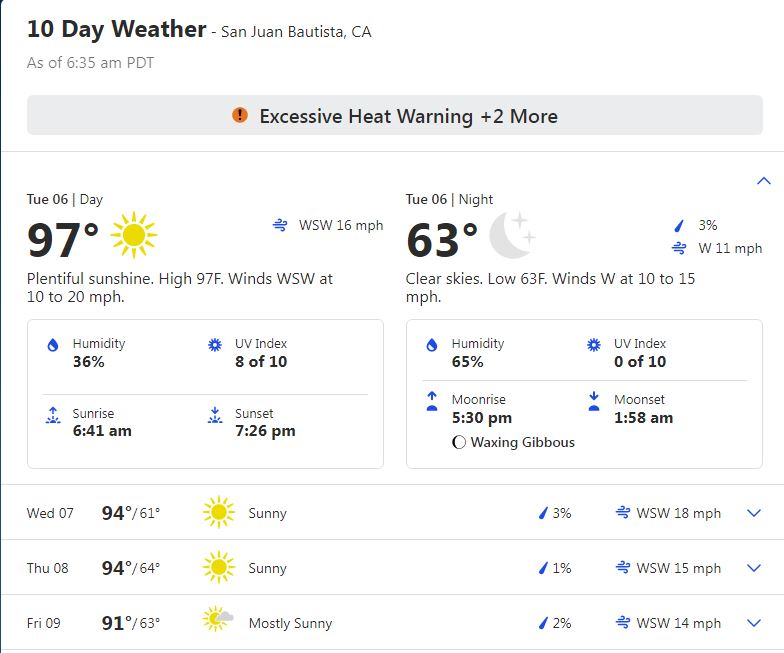**10-Day Weather Forecast for San Juan Bautista, California (as of 6:35 a.m. PDT)**

Current Conditions: An excessive heat warning is in effect along with two additional weather alerts.

**Tuesday, June 6**:
- **Daytime:**
  - Temperature: 97°F
  - Weather: Plentiful sunshine
  - Winds: West-southwest at 10 to 20 miles per hour
  - Humidity: 36%
  - UV Index: 8 out of 10
  - Sunrise: 6:41 a.m.
  - Sunset: 7:26 p.m.

- **Nighttime:**
  - Temperature: 63°F
  - Weather: Clear skies
  - Chance of precipitation: 3%
  - Winds: West-southwest at 10 to 15 miles per hour
  - Humidity: 65%
  - UV Index: 0 out of 10
  - Moonrise: 5:30 p.m.
  - Moonset: 1:58 a.m.
  - Moon Phase: Waxing Gibbous